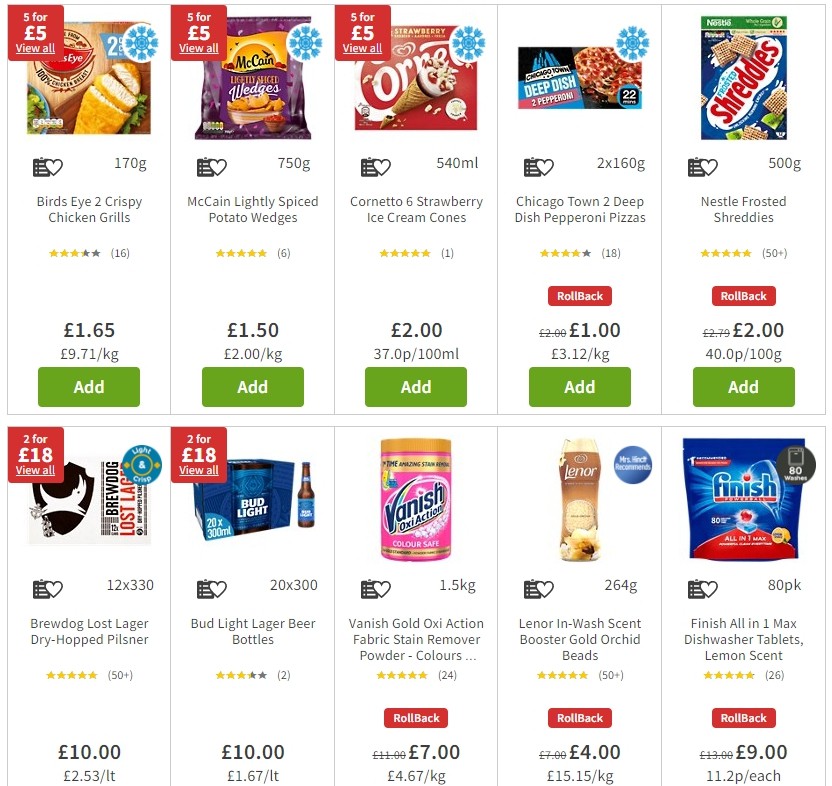Screenshot of a grocery website featuring ten different products. The top left corner displays Bird's Eye Crispy Chicken Browns, accompanied by an image and a deal offering five for five pounds, with an option to view all related items. Next is McCain Lightly Spiced Potato Wedges, similarly priced at five for five pounds, and also offering the view all option. Following this, there's a picture of six Cornetto Strawberry Ice Cream Cones. Further down, there's an image of Chicago Deep Dish Pepperoni Pizza, and a box of Nestlé Frosted Shreddies.

On the subsequent row, BrewDog Gloss Lager and a box of Bud Light are shown. Additionally, there is a container of Vanish Gold Oxy Action Fabric Stain Remover Powder Colors. The lineup continues with Lenor's In-Wash Scent Booster Gold Orchid Beads and concludes with Finish All-in-One Max Dishwasher Tablets in a lemon scent. Each product is accompanied by its respective image and deals or descriptions pertinent to the item.